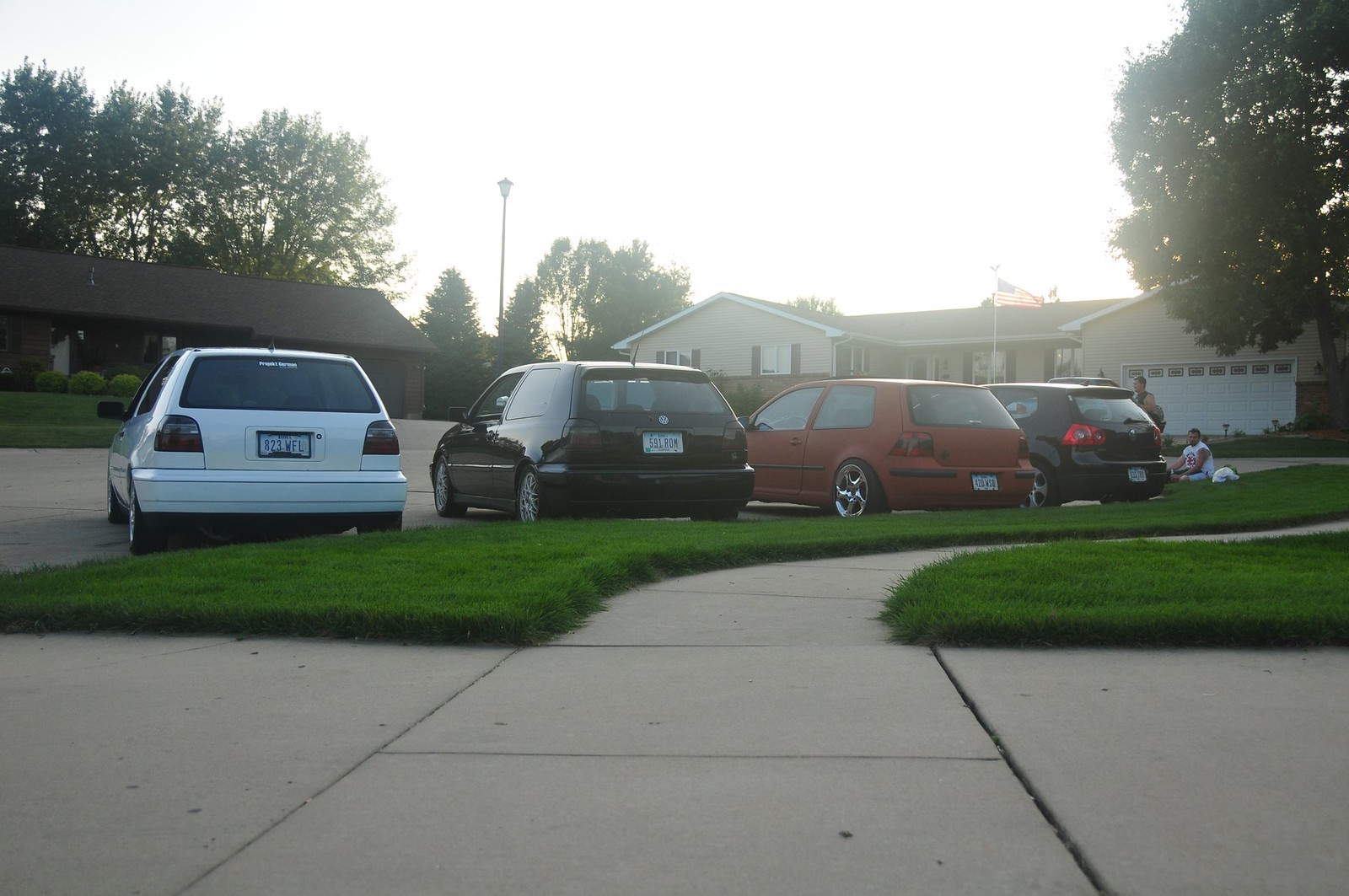In this suburban American neighborhood scene captured during dusk, we see a row of four Volkswagen Golf cars (white, black, red, and black) parked in a cul-de-sac. The compact sedans appear to be slightly modified, with the red one featuring silver rims. The cars are oriented away from us, revealing their license plates and back sides. On the sidewalk at the end of the cul-de-sac, two people, one in a sleeveless white t-shirt, are accompanied by what seems to be a dog. The background showcases an off-white house with a prominent white garage and an American flag, flanked by a large tree on the right. To the left, a brown house with a dark roof is partially obscured by another bank of trees. The bright sky appears washed out from the sun, adding to the serene dusk atmosphere of this well-kept suburban setting.